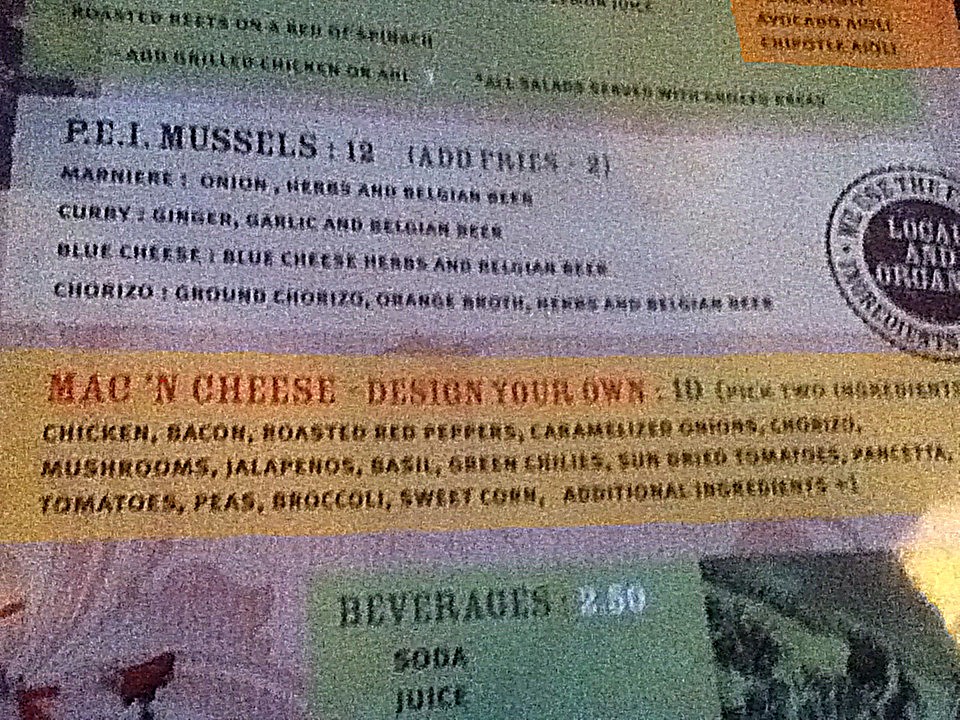The photograph captures a close-up of a heavily blurred and grainy menu. The menu design features horizontal stripes in olive green, light blue, and orange. Despite the poor image quality, the following details could be discerned:

- The central section of the menu highlights a dish titled "PEI Mussels," which is priced at $12. An additional note indicates that fries can be added for $2. 
- Adjacent to this section, a small circular symbol is partially visible, likely reading "local and organic," though the word "organic" is cut off. 
- In the orange stripe below, there's an item labeled "Mac and Cheese," allowing for customization, with a base price of $10. It is followed by a list of available ingredients for personalization.
- The bottom portion of the menu features a green rectangle that lists beverages such as soda and juice, though the text is truncated.

Additionally, the lower part of the image appears to include a nature-themed photograph, although details are indiscernible due to the graininess. A light reflection is noticeable in the bottom right corner, further obscuring the image.